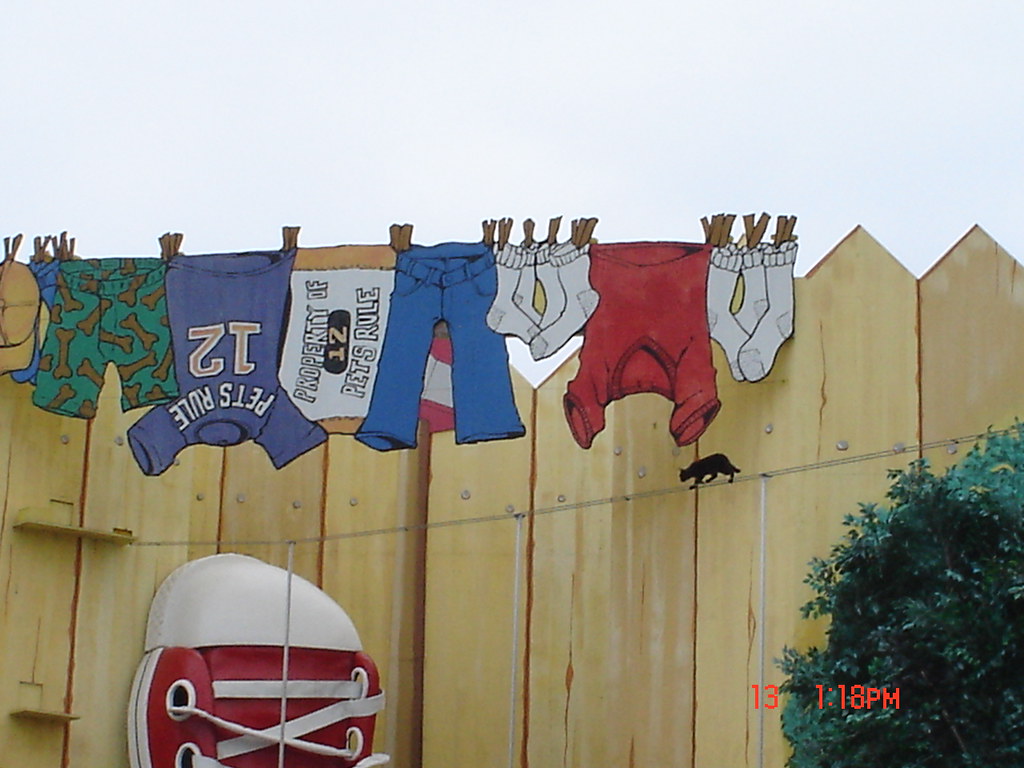In this intriguing outdoor photograph taken on the 13th at 1:18 PM, a medium-colored wooden fence with pointy-tipped posts spans the background, with no gaps between the pickets. A large, red and white plastic sneaker, resembling a Chuck Taylor, is prominently displayed atop the fence. Below the sneaker, a green bush occupies the lower right corner of the image. Along a horizontal rope strung on the fence, a small metal silhouette of a black cat is seen walking. Above this, a whimsical array of cartoon-drawn laundry hangs from wooden clothesline clips: white socks, a red t-shirt, blue jeans, a jersey inscribed with "Pet’s Rule #12," and teal green shorts adorned with brown dog bone images. The surreal blend of real elements and cartoon artwork creates a captivating visual narrative.